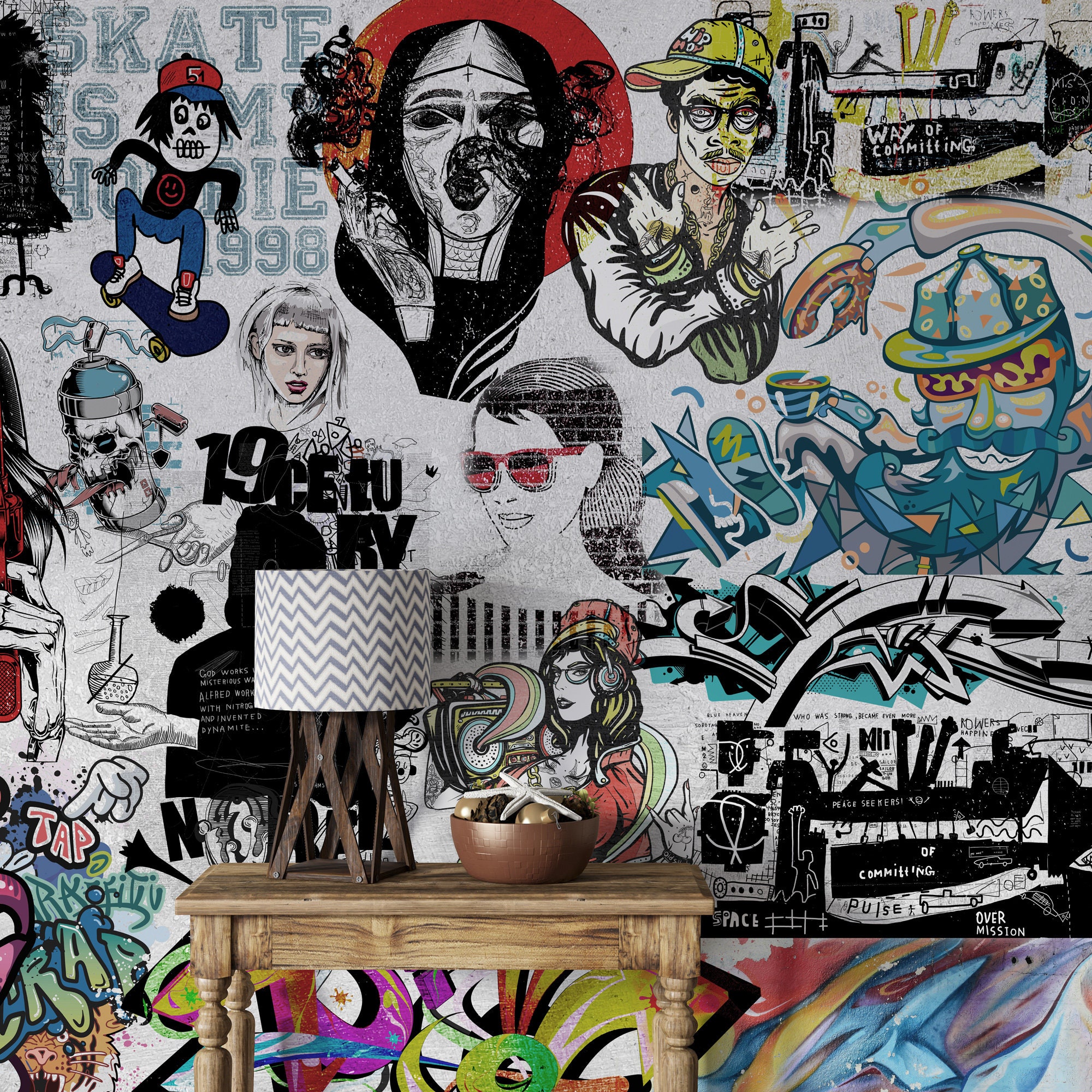The image features a vibrant and eclectic wallpaper brimming with urban, youthful energy, reminiscent of street art and personal expression. Dominating the background are scenes of graffiti-like artwork in various hues of purples, greens, yellows, reds, blues, pinks, lime green, black, white, and teal. The wallpaper's details include a skeleton-faced boy on a skateboard, women wearing headphones, a gentleman with a sideways baseball cap making peace signs, and a smoking woman, all mingled with graffiti-like texts such as "skate is my hobby" and "Tap and Wrap." In the upper left corner, a partial reference to the year 1998 is visible. In the foreground sits a natural wooden table featuring a lamp with a gray and white sawtooth patterned shade supported by an X-shaped frame, and a round bowl containing acorns, muted gold-hued bulbs, a starfish, and what might be popcorn. The dynamic artwork flows beneath and around these objects, creating an immersive and visually stimulating scene bursting with individuality.